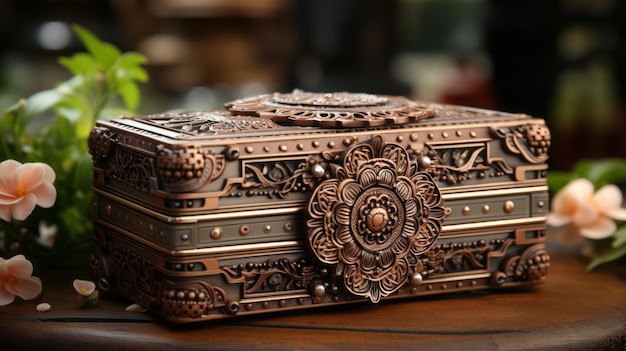This professional photograph showcases an exquisite, ornately carved jewelry box positioned on a rounded wooden tabletop. The box, which exudes a steampunk aesthetic, has a dark bronze or coppery hue with intricate detailing throughout. The central focus includes intricate floral designs, notably a large medallion on the top and a prominent flower-like emblem on the front, which may also serve as a clasp. Every inch of the box is adorned with elaborate patterns of ridges, dots, swirls, and ivy motifs, contributing to its luxurious and expensive appearance.

A band painted in olive green runs around the box, bordered by gold edges, studded with evenly spaced small circles of varying sizes. The medallion and floral designs are echoed on the top and sides of the box, enhancing its ornate quality. The setting includes several peach-colored flowers, likely geraniums, and accompanying green foliage, which though partly blurred, add beauty and depth to the background, reinforcing the box’s focal prominence and luxurious allure.